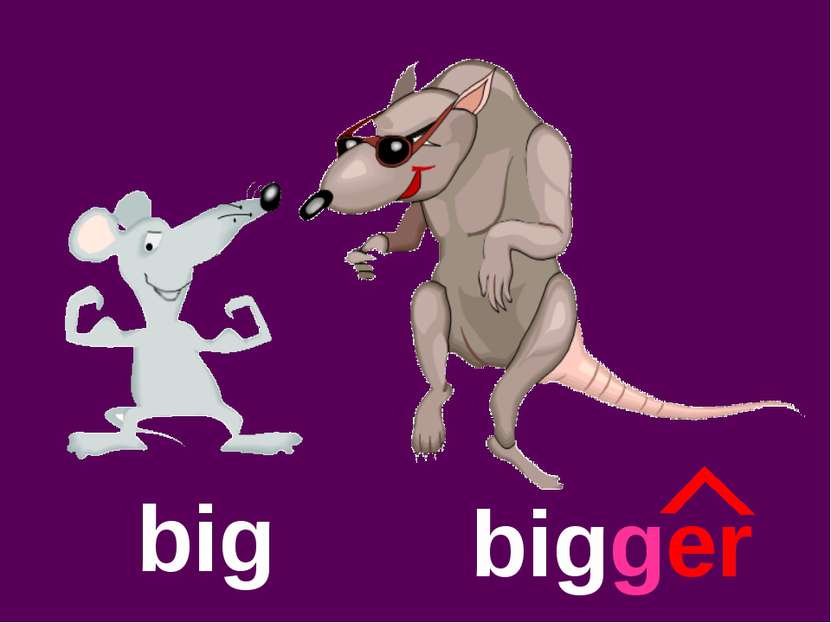Against a dark purple background, an image depicts two anthropomorphic rodents with contrasting sizes and expressions. On the left, a smaller, bluish-gray mouse stands confidently, flexing its prominent biceps with its feet spread apart, pointing away from each other. Its large head is topped by a black nose and whiskers, and one eye gazes directly at the viewer with a cheerful smile. Below this mouse, the text "big" is written in lowercase white letters.

To the right, a much larger, menacing rat stands taller with a dark greenish-gray body and pointed ears. Wearing dark sunglasses and sporting a red, smiley mouth, the rat appears to be mid-tiptoe dance, with one back paw raised and arms bent at the elbows. Its long, fleshy tail extends out to the right. Below this imposing rat, the layered text reads "bigger" in a mix of white and red lowercase letters, with a stylized triangular frame above the "er" part of the word.